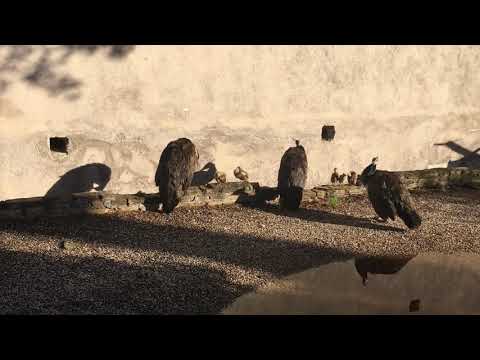In the image, three large vultures are seen standing and pecking at a gravel-covered ground, their dark, featherless heads and necks prominently visible. The setting appears to be an outdoor area during the middle of the day, evidenced by the bright sunlight casting distinct shadows of the vultures and other objects. A small puddle is located in the bottom right corner of the photo. They are positioned almost centrally in the image, with one vulture on the left, one in the center, and one on the right, two of which are perched on a low wooden rail running horizontally across the middle of the frame. The backdrop reveals a beige-grey cement wall with two square cutouts, near which the birds' shadows are noticeably cast. There is also a small green tuft of plant life emerging from the ground towards the right side of the image. The earthy tones of black, white, various shades of grey, and tan dominate the color palette, with very minimal greenery observed.